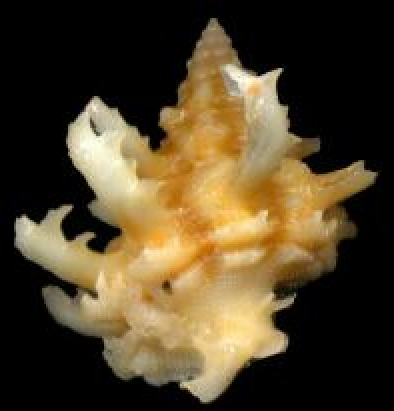The photograph features a detailed close-up of a seashell against a solid black background. The seashell showcases an intriguing combination of warm colors, ranging from brown and orange to manila-white and hints of gold. It has a distinctive, conical top that narrows into a needle-like point, reminiscent of a screw. The surface of the shell is textured with ridges and edges, and it is adorned with jagged, prong-like protrusions that are both sharp and rounded in different areas. The simplicity of the background draws full attention to the intricate details and colors of the seashell, making it the central focus of the image. This seashell, possibly once home to a snail, captivates with its rugged and uniquely-formed exterior.